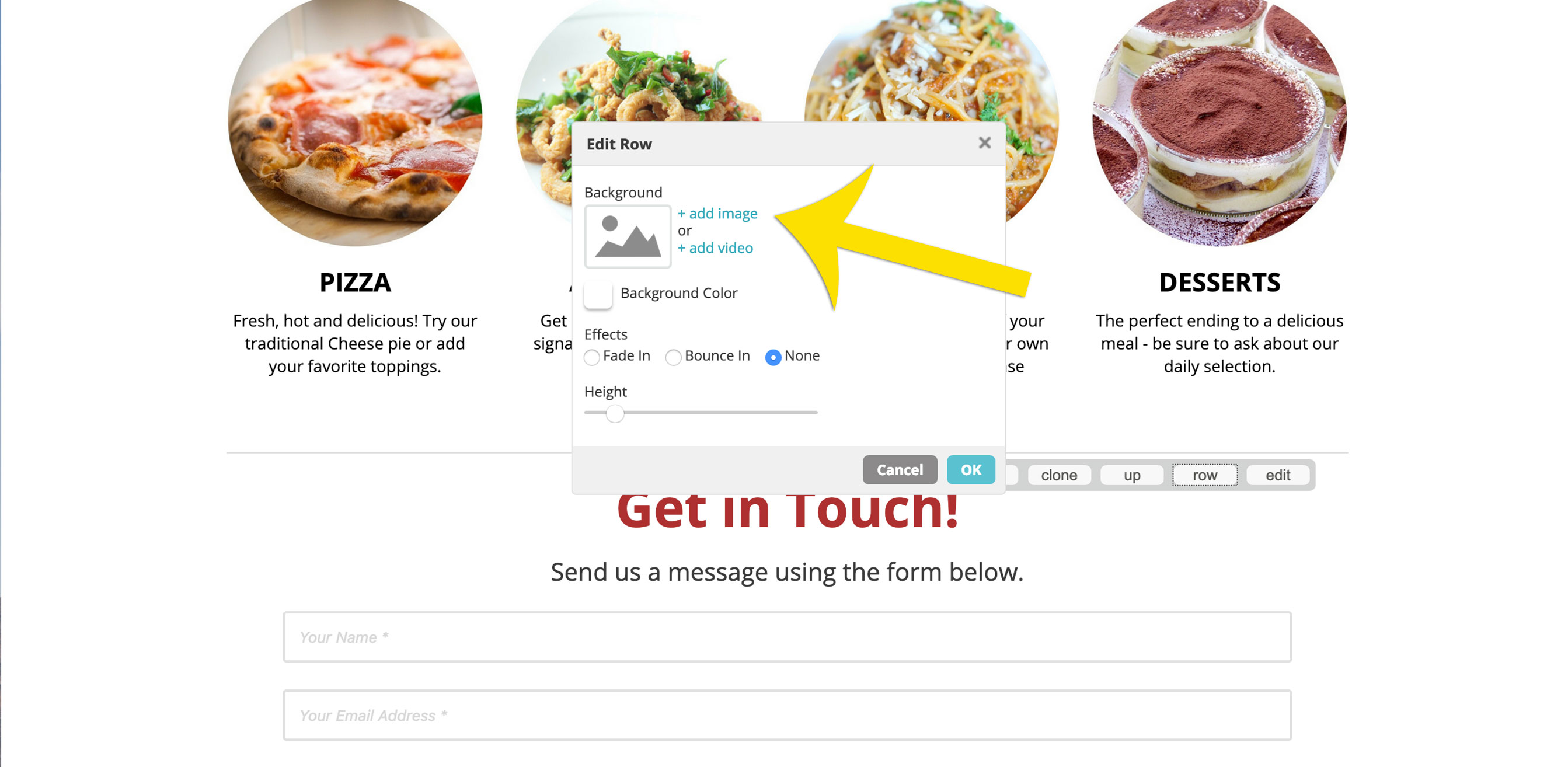This is an image set against a completely white background, prominently featuring a horizontal arrangement of four food pictures across the upper half. 

1. **Top Left**: 
   - **Image Description**: A sumptuous pizza adorned with pepperoni slices and various other toppings.
   - **Caption**: "Pizza: Fresh, hot, and delicious. Try our traditional cheese pie or add your favorite toppings."

2. **To the Right of the Pizza**:
   - **Image Description**: Crispy onion rings garnished with green herbs.
   - **Caption (part of the general layout)**: Included indirectly as food item details.

3. **Next to the Onion Rings**:
   - **Image Description**: A delectable serving of noodles, sprinkled with green herbs and white cheese.
   - **Caption (part of the general layout)**: Detailed above under "pizza" and indirect text.

4. **Farthest Right**: 
   - **Image Description**: Tempting assortment of cakes or desserts.
   - **Caption**: "Desserts: The perfect ending to a delicious meal. Be sure to ask about our daily selection."

The central part of the image is obscured by an editing interface box, which is aligned vertically and displays the following options:
   - **Left Side of the Box**: "Edit Row", "Background"
   - **Right Side of the Background Section**: Buttons labeled "Add Image" and "Add Bids" in blue letters, below which are options for "Background Color" and "Effects". Within "Effects", "None" is checked, accompanied by a height adjustment bar.
   - **Bottom Right of the Box**: Buttons labeled "Cancel" and "OK".

Below this box:
   - **Text in Red**: "Get in touch"
   - **Followed by Black Text**: "Send us a message using the form below."
   - **Below the Text**: Two lines or fields intended for users to send their messages. 

This organized layout effectively showcases food offerings while incorporating editable interface elements for better user interaction.